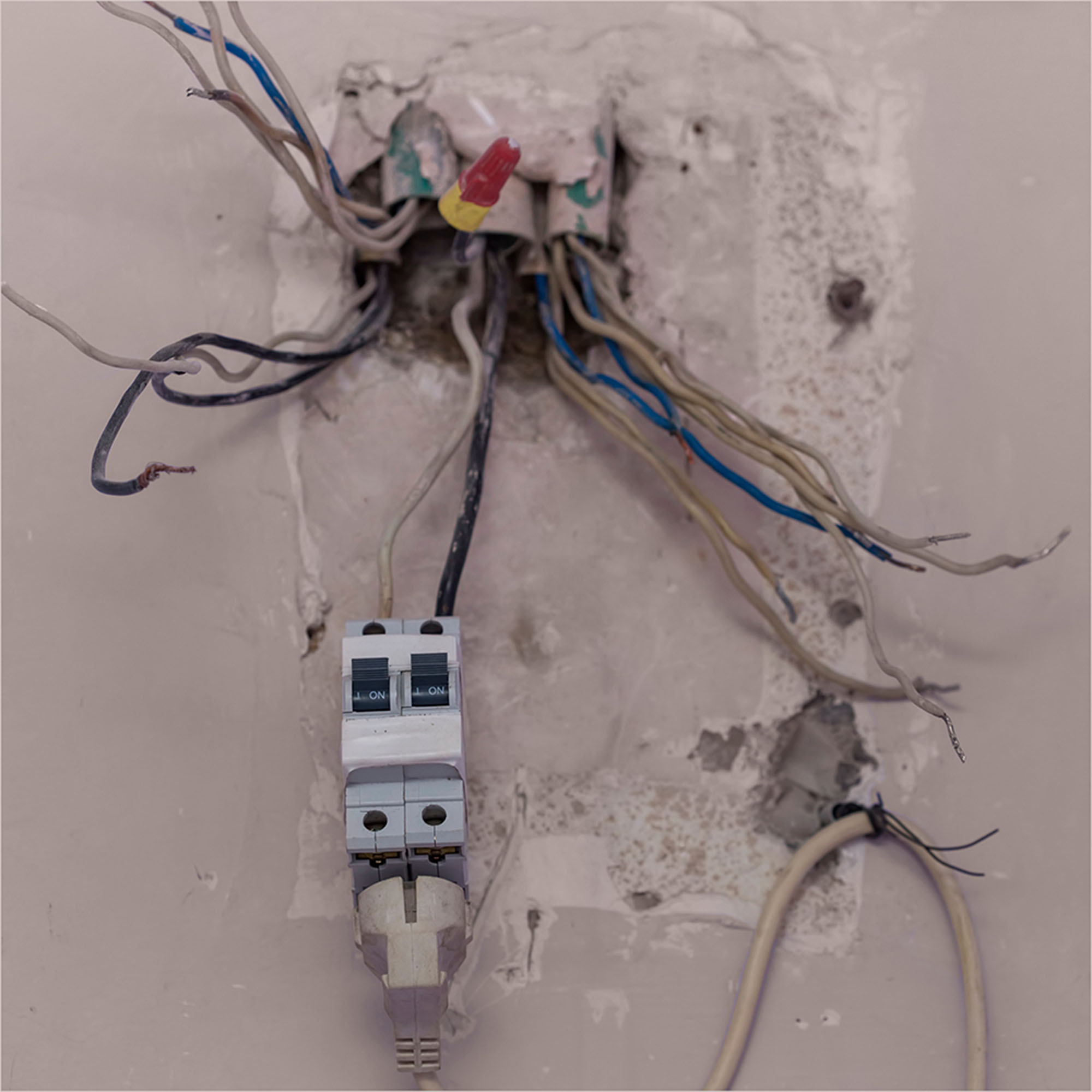The image depicts a heavily damaged electrical system with exposed wiring protruding from a gray wall. Multiple sections of cables—blue, brown, black, white, and gray—are visible, likely numbering between three to six distinct segments. Some wires have caps, including a black wire with a yellow and white cap. Additionally, certain wires appear to be aged and potentially cut or disconnected from whatever they were originally attached to, indicating a need for repair. Holes and gaps suggest that a cover or protective plate has been removed or has fallen off. Among the mess, a European-style plug remains connected to an outlet, which has an on-off switch and looks precariously zip-tied to the wall. The overall scene highlights safety concerns and an urgent need for professional electrical repair.